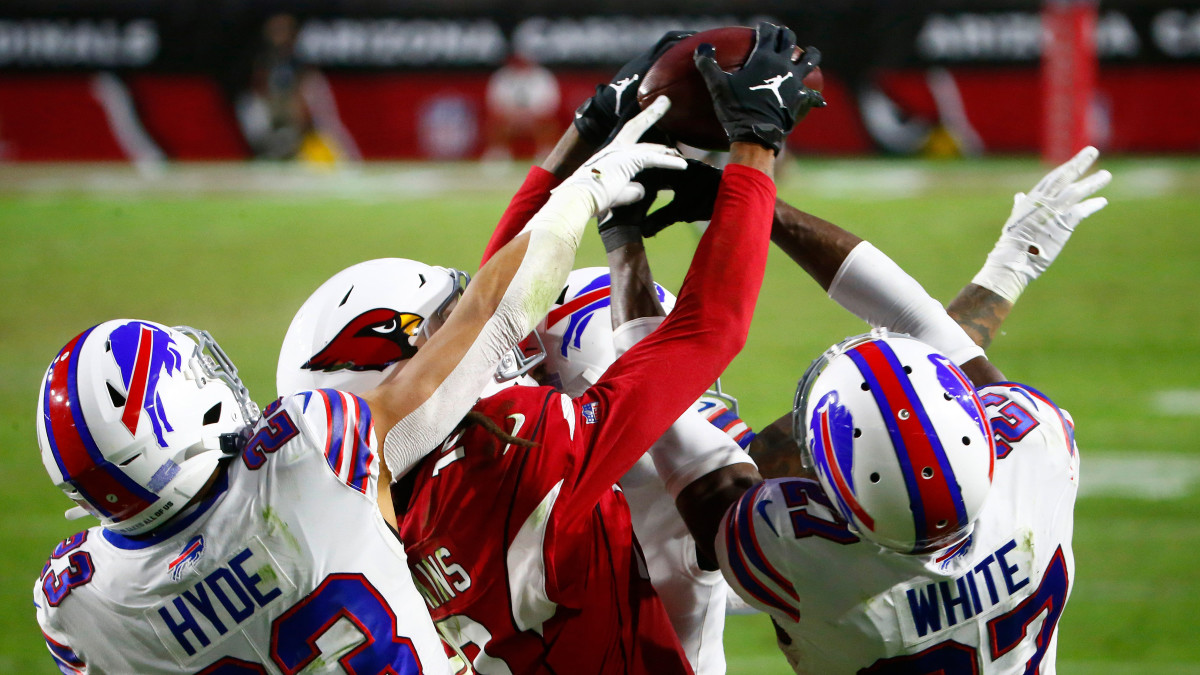This vivid photographic freeze-frame captures the intense moment of an American football game. At the heart of the image, four players are captured mid-air, all striving to grasp the football. The central player, donning a red jersey with white numbers, is from a team whose helmet displays a cardinal logo. This player, gloved in black, securely clutches the ball while looking upwards toward it. Flanking him are players from the opposing team, who sport white jerseys with blue and red numbers, and white helmets featuring a red stripe and a buffalo logo. The players identified by their jerseys are Hyde on the left and White on the right, each reaching out for the ball. Another teammate in white is partly visible in the back. The scene unfolds over the vibrant green of the football field, set against a backdrop of out-of-focus stands, predominantly red, adding to the dramatic tension of the moment.